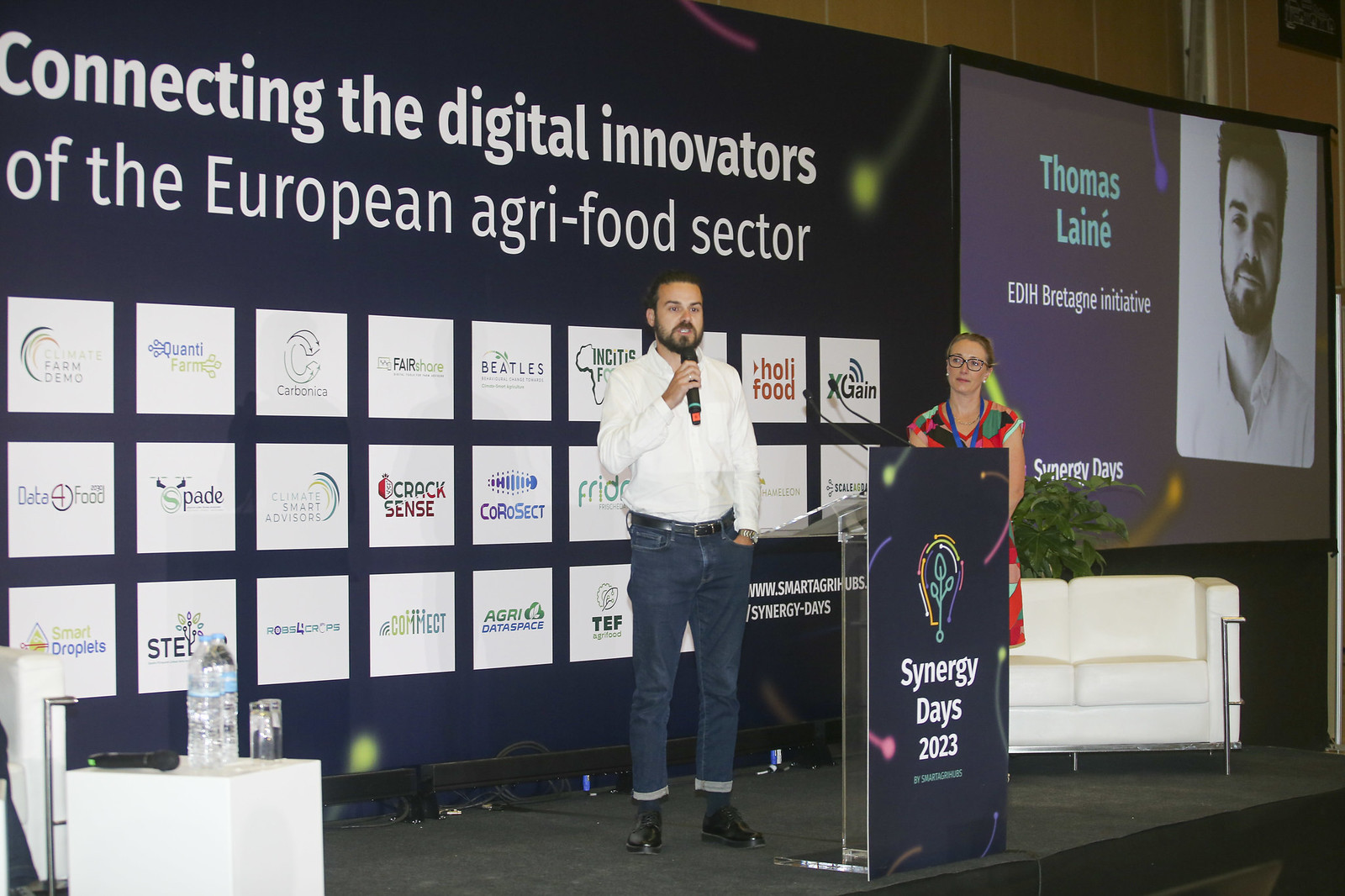The horizontally aligned rectangular image captures a stage setup at a convention themed around the European agri-food sector. Center stage, a man with short brown hair and brown facial hair holds a microphone while speaking, dressed casually in cuffed blue jeans, a white button-down shirt, a black belt, and black boots. He stands behind a clear lectern adorned with a sign that reads "Synergy Days 2023" in white text, featuring a stylized multicolored light bulb with three leaves in place of filament. 

To his side, a woman in glasses, with her hair pulled back into a ponytail or bun, listens attentively. She wears a vibrant orange-patterned dress with red and green elements and a blue lanyard, standing near a white loveseat partially visible in the background. 

Behind the speakers, a large banner prominently displays the message "Connecting the Digital Innovators of the European Agri-Food Sector" in white text. Adjacent to this on the right side of the stage is a screen showing a black and white photo of a man identified as Thomas Lane, labeled as part of the "EDIH Britagny Initiative." The backdrop also features a collection of square papers showcasing sponsors' names and logos, including Spade, Cracksense, Corosact, The Beetle, Fair Share, Smart Droplets, and Delta Food.